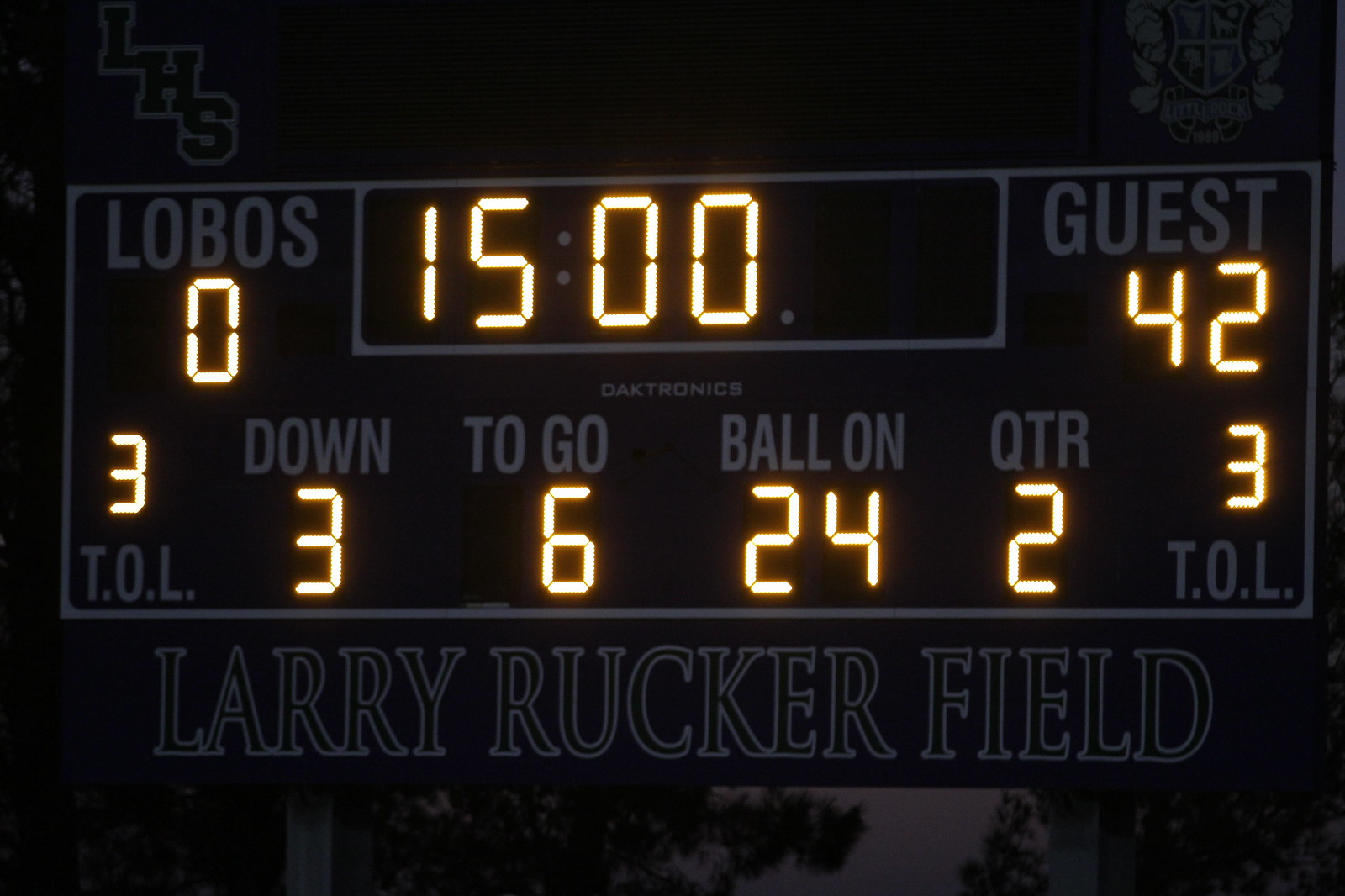This horizontally aligned rectangular photograph captures a detailed image of a navy blue scoreboard, likely situated at a high school sports field, against a dark, nighttime sky. In the upper left-hand corner, the letters "LHS" are prominently displayed in black and outlined in gray, while the upper right-hand corner features a royal crest-like team logo. The central portion of the scoreboard is dominated by a large, horizontal rectangle labeled "Lobos" on the left and "Guest" on the right. The scores are lit up with LED lights: "Lobos" with an orange or yellow 0 and "Guest" with 42. Between these team names, the time is indicated as "15:00." Below this, a series of lit-up indicators provide game-specific details: "TOL" with a 3 above it, "Down" with a 3 below it, "To Go" with a 6 below it, "Ball On" with a 24 below it, and "QTR" with a 2 below it. The lower right-hand corner also displays "TOL" with another 3 above it. The bottom section of the scoreboard prominently features "Larry Rucker Field" in large, all-capital letters. Additional details include a gray outline and branding text "Daktronics" in the middle. The overall minimal lighting accentuates the vivid scoreboard against the dark background.